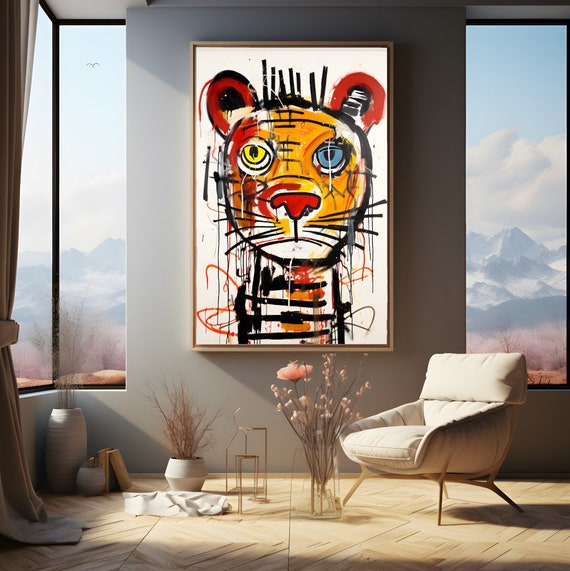In the image, we observe a sunlit room with a pale wood floor. On the right side towards the bottom, there is a beige chair with cushions. Centrally and at the bottom of the image, a vase filled with pink flowers, affixed to long brown stems, dominates the scene. To the left of this vase, another pot with brown branches can be seen, with a beige cloth piled in front of it. Further left, there are additional pots, and a curtain drapery extends from the bottom left of the image to the top, partially concealing tall windows that span the left side, middle, and top left of the image. Moving to the center and top middle of the image, a painting on a gray wall depicts a seemingly abstract, low-resolution tiger with black stripes. On the right side of the image, another tall window offers a view of mountains, blue skies, and clouds. The scene features a variety of colors, including red, orange, yellow, black, beige, tan, blue, light blue, brown, gray, and pink, and it captures a real, daytime photograph taken at eye level, possibly from a standing position.